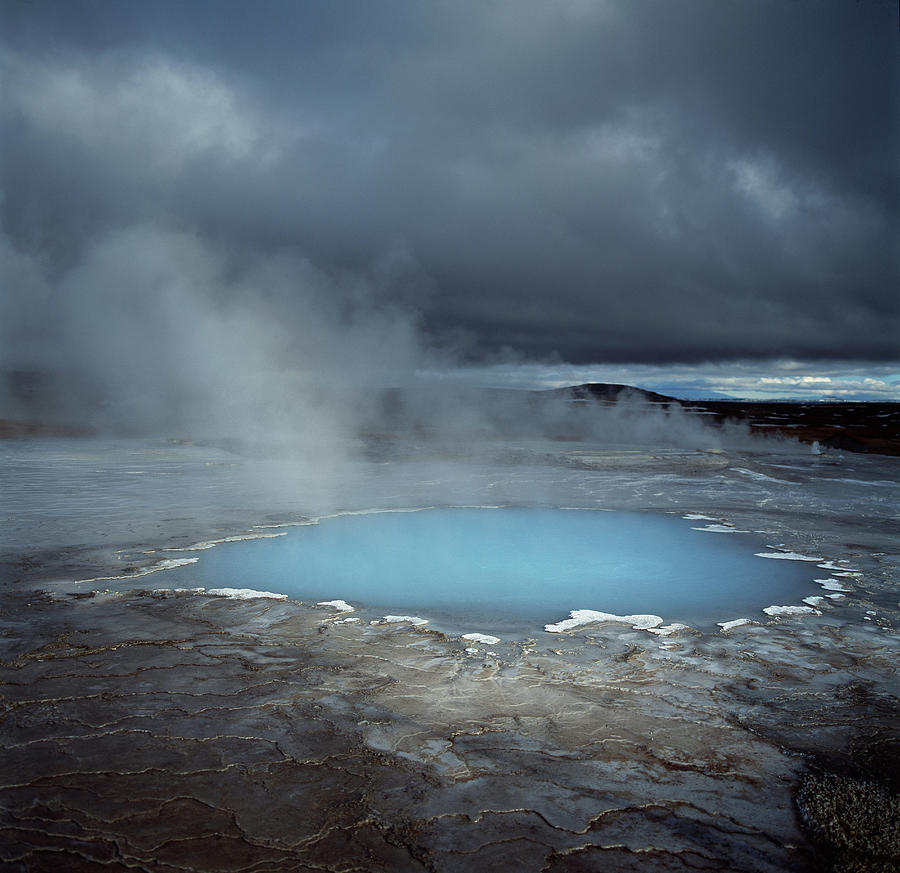The square photograph captures an expansive outdoor setting, framed by a dynamic sky where thick grey clouds dominate the upper portion, but reveal patches of vibrant blue and white clouds further back. Central to the image is a bright blue body of water, likely a hot spring, emitting visible steam that creates an ethereal atmosphere. This hot spring is surrounded entirely by a rugged, grey rocky terrain with noticeable white areas along the water's edge, possibly from mineral deposits. The rocky surface appears hard-packed and somewhat flaky. In the distant background, a faint hill is visible beneath the cloud-covered sky, reinforcing the sense of vastness and solitude in this striking landscape.